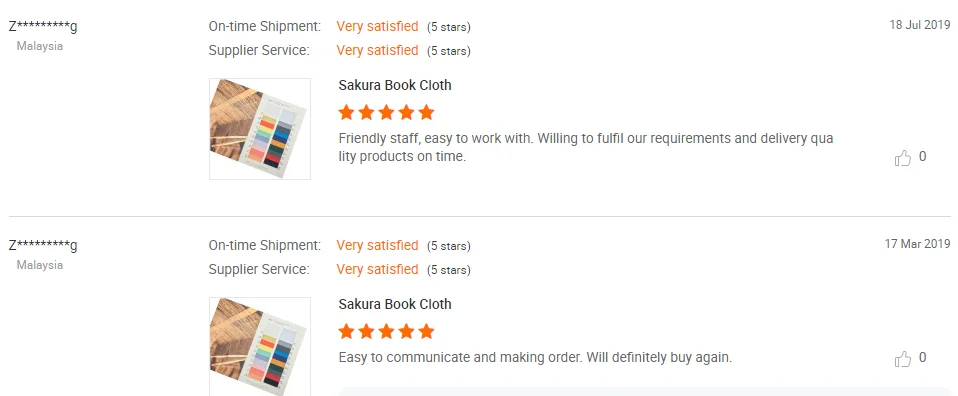Sure, here is a cleaned-up and highly detailed descriptive caption for the given image:

---

**E-commerce Product Review Summary**

This screenshot captures a section of user reviews for a product listed on an e-commerce site. Notable elements include the absence of purchasing options in this specific view. The key details are as follows:

1. **Seller Information:**
   - **Name:** Redacted (starts with 'Z' and ends with 'G').
   - **Location:** Malaysia.
   - **Same name for both review entries.**

2. **Review Highlights:**
   - **Ratings:**
     - **On-time Shipment:** "Very Satisfied" with a five-star rating, displayed in orange.
     - **Supplier Service:** "Very Satisfied" with a five-star rating, displayed in orange.

3. **Product Details:**
   - **Sakura Book Cloth:**
     - Featured image showing a possibly wooden beam ceiling.
     - Noted with a five-star review.
     - Positive feedback: "Friendly staff, easy to work with, willing to fulfill our requirements and deliver quality products on time."
   - **Review Date:** 18th July 2019.
   - **Thumbs-Up Selection:** Zero thumbs-up.

4. **Additional Review:**
   - **Sakura Book Cloth:**
     - Consistent with the previous details and image.
     - Identical five-star rating and positive feedback highlighting ease of communication and satisfaction with order fulfillment.
   - **Review Date:** 17th March 2019.
   - **Thumbs-Up Selection:** Zero thumbs-up.

**Note:** This screenshot primarily showcases user feedback and ratings, without direct links or buttons for purchasing the product.

---